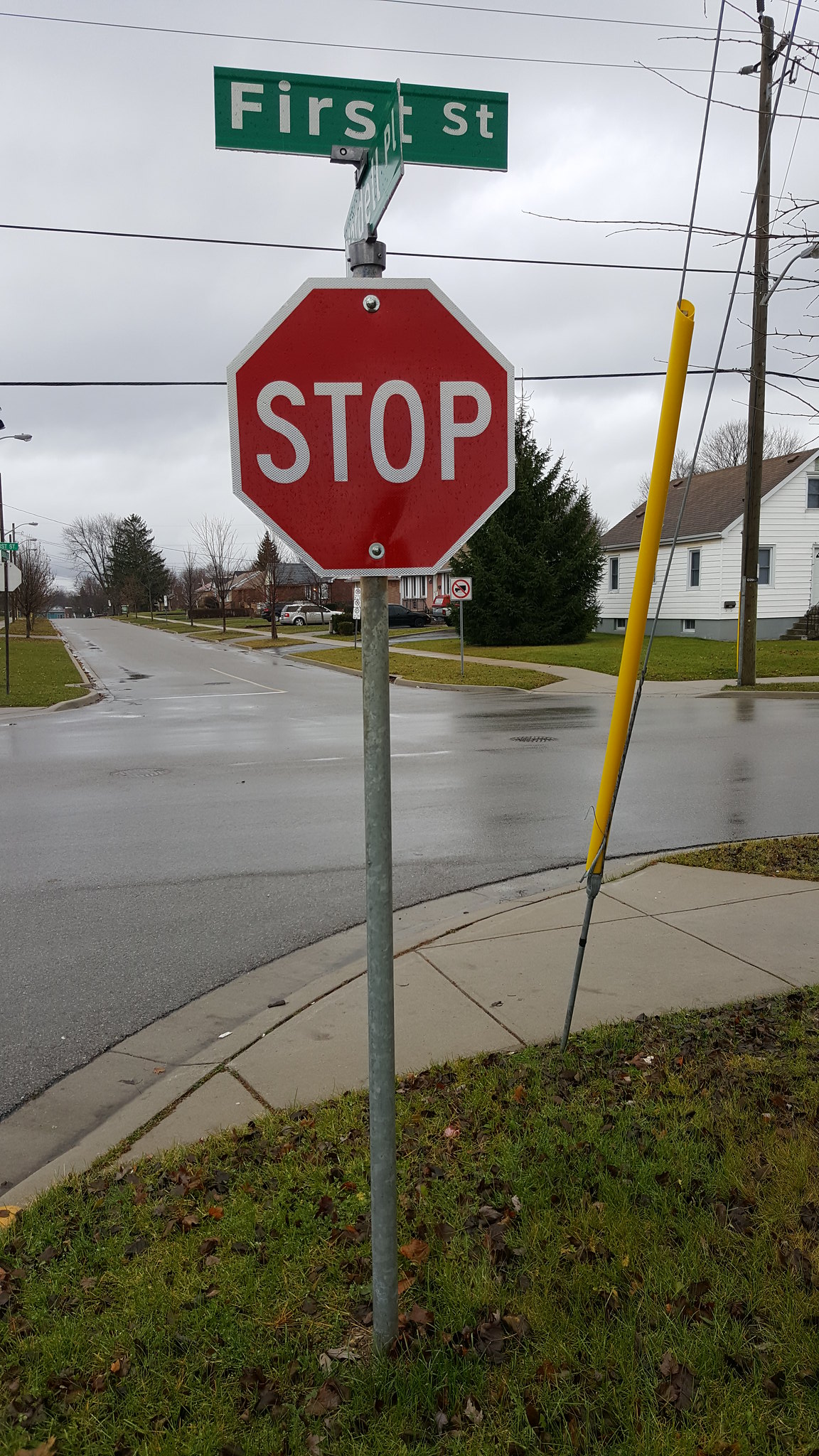The photograph captures a rain-soaked suburban intersection, dominated by a classic red and white octagonal stop sign mounted on a grey metallic pole. Atop this pole are green street signs with white text; the visible one reads "First Street" (F-I-R-S-T), while the intersecting street sign is partially obscured but ends with “Place”. Several yellow-sheathed cables, likely for power line stabilization, extend tautly from the ground. The backdrop reveals a mix of wooden slatted and brick homes, all featuring steep, A-frame roofs. Drenched streets with shallow curbs and heavy, dark skies complete the scene, emphasizing the recent downpour. A nearby sidewalk and scattered vehicles further enhance this quintessential American suburban vista.